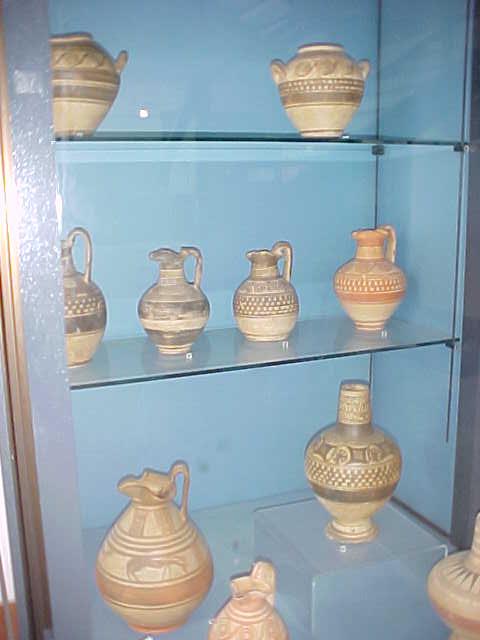This photograph captures a light blue display cabinet with a glass front, likely taken with a flash as indicated by the reflection in the top left, where the polished wooden frame reflects the light. The cabinet features two glass shelves and a bottom shelf, all lined with ancient-looking pottery that could easily be mistaken for artifacts from a museum or something you'd see on the History Channel.

The cabinet's interior, including the back and side walls, is painted pale blue, which contrasts with the glossy, brown-tinted wood of the frame. Each shelf hosts a collection of clay vessels, including urns, ewers, jugs, and pitchers, all adorned with intricate bands of designs - such as animals, geometric patterns, or simple stripes. The color palette of these artifacts ranges from gray to pale brown, with some featuring reddish hues, highlighting their age and possible ancient origins.

On the top shelf, there are two rounded urns with small handles, decorated with horizontal darker brown lines. The middle shelf contains various jugs characterized by their rounded bodies, spouts, and handles, painted in earthenware tones, with one distinctly more reddish than the others. The bottom shelf holds larger jugs and urns, some of which depict figures, like a horse, against the fawny brown-beige backdrop with red and brown highlights.

Overall, the photograph, despite the slight overexposure from the flash, clearly showcases these historically styled vessels, capturing their intricate details and reflective display in a well-lit, organized setting.